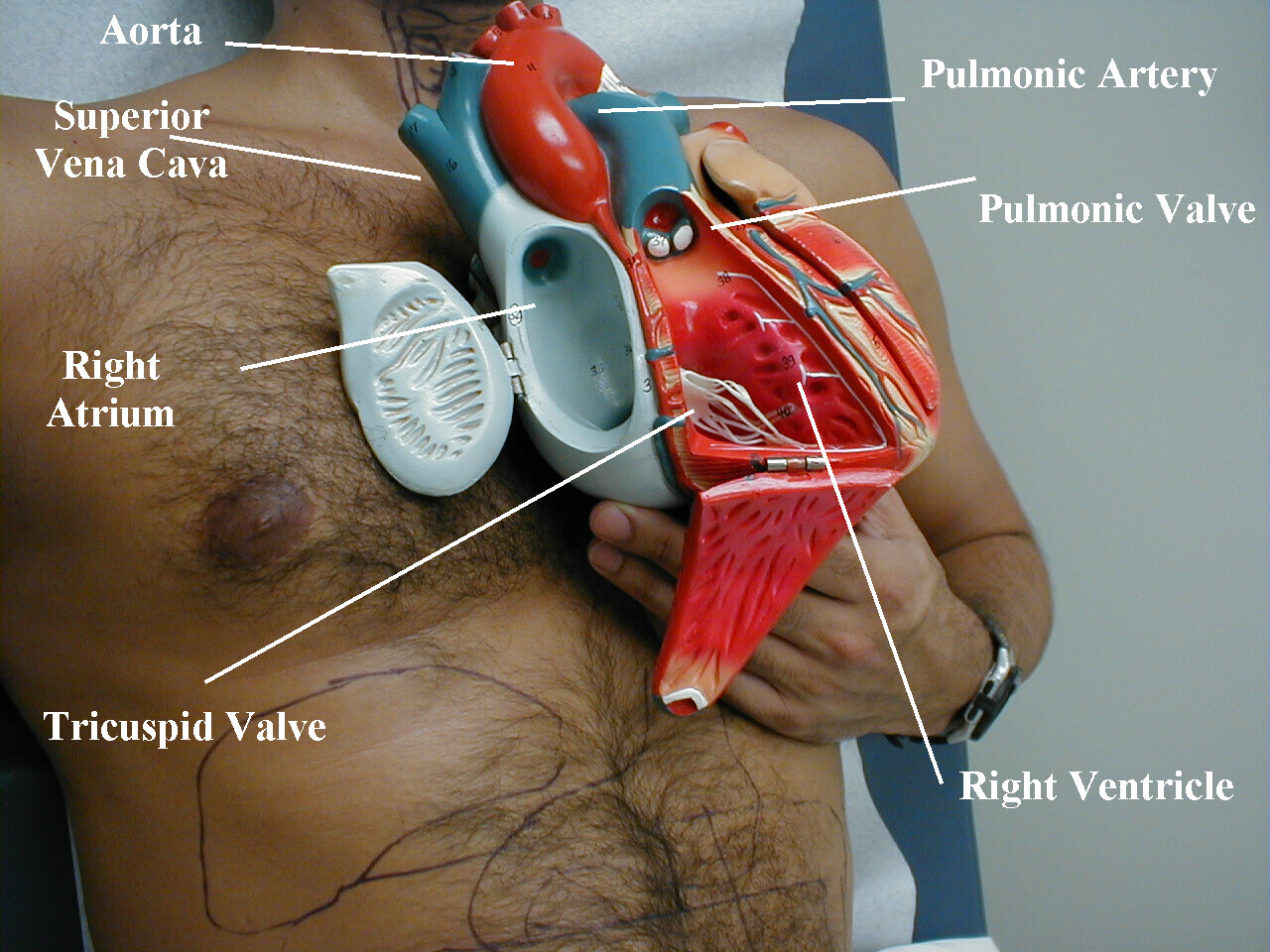The captivating image portrays a middle-aged, shirtless man with chest hair, lying on a medical bed while holding a large, detailed plastic replica of the human heart against his chest. This stark and slightly surreal scene is set in an array of colors—primarily brown, red, and blue, with hints of green and gray. The heart replica, depicted with vivid, graphic precision, displays labeled anatomical parts such as the aorta, pulmonary artery, pulmonic valve, right atrium, right ventricle, and tricuspid valve in white text. The background and overall composition suggest a medical setting, likely designed for educational purposes, reminiscent of a poster one might find in a doctor's office. This instructional image melds a raw, humanized element with clinical detail, effectively highlighting the intricate workings of the heart.